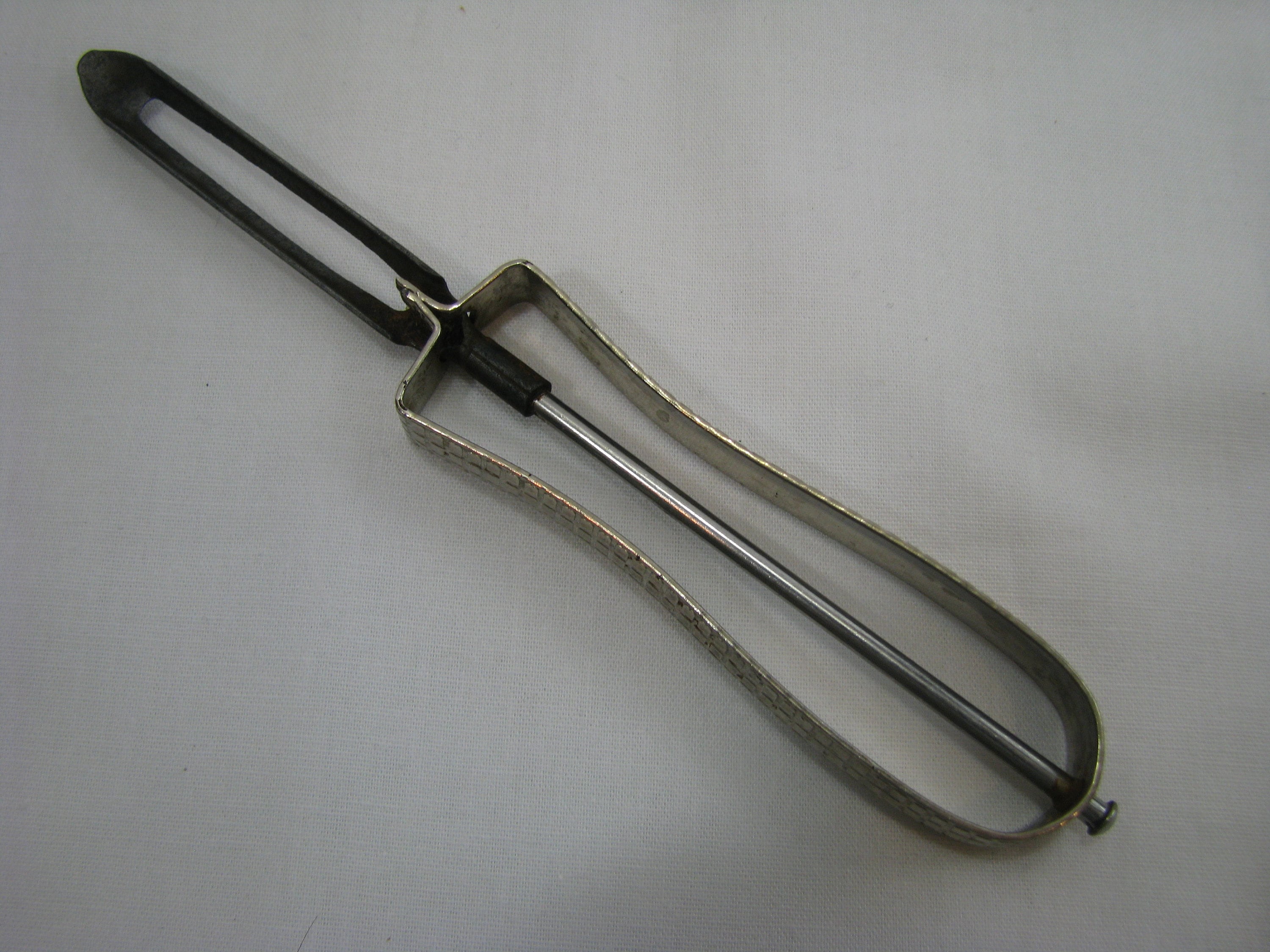A detailed image depicts a metal vegetable peeler resting on a gray surface. The peeler features a black handle positioned in the upper left corner that curves down to the right, reminiscent of a long, pill-shaped cucumber. The handle connects to a top and bottom piece, forming an elongated oval structure with a space in between, slightly fuller at the top, tapering down to a metal component. This component spreads out to the left and right, curving inward slightly before extending outward again, and then rounding off at the bottom. Running the length of the device, a small, black cylindrical piece in the middle merges with a silver cylindrical post, terminating in a disc-like knob. The peeler includes a sharp, indented blade within the hollow oval section, designed for peeling vegetables such as potatoes or cucumbers. The scene is set against a light purplish-gray background that may be a fabric or board surface.